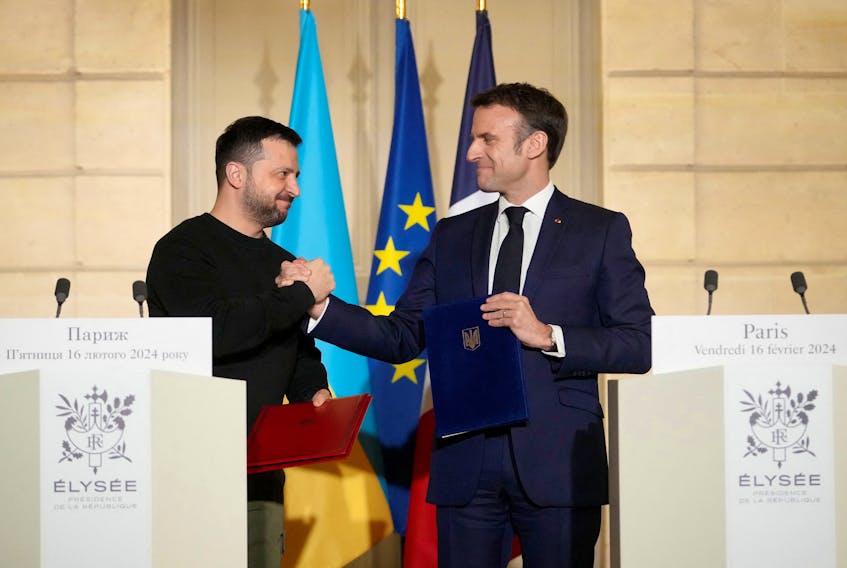The image captures a formal moment between two presidents, the President of Ukraine on the left and French President Emmanuel Macron on the right, as they shake hands firmly, almost gripping each other's fists in a gesture that could signify congratulations or mutual respect. To the side of each president stands a podium; on the right podium, marked with "Paris" and the date "16th of February, 2014," there's a crest that reads "Elysee." The left podium also has the word "Elysee," and features text in Russian. The President of Ukraine is dressed in a dark long-sleeved t-shirt and holds a red book, while President Emmanuel Macron wears a navy blue suit paired with a white shirt and navy blue tie, holding a navy blue book. Behind them, three different flags are displayed: one light blue, another darker blue with a yellow star design, and a navy blue flag, symbolizing their respective countries. The pulpit features the text "Paris, May 16, February 24," along with the acronym "LEC."